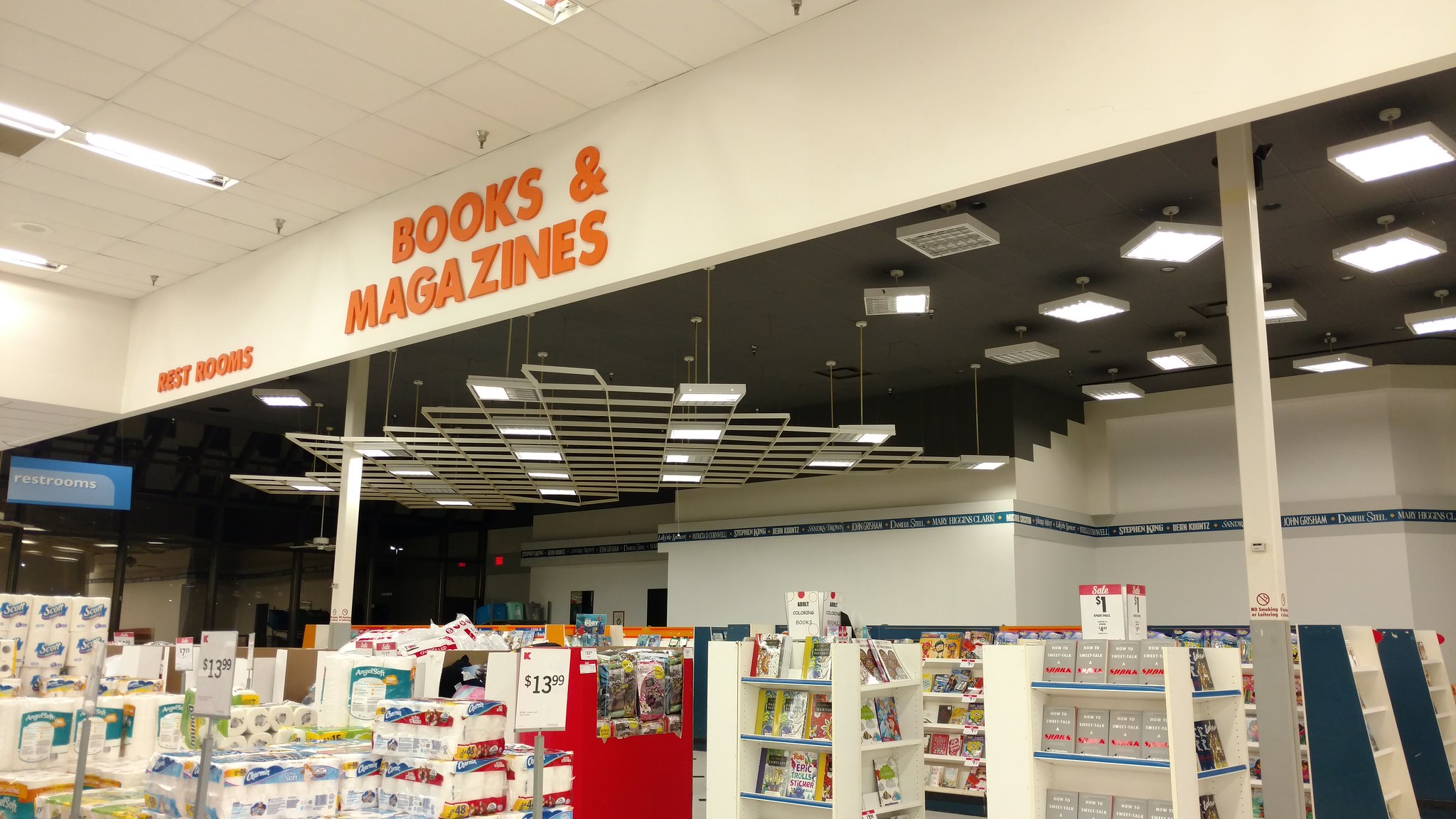The image depicts the interior of a mixed-goods store featuring both household items and reading materials. Prominently displayed at the front are multiple stacks of toilet paper and paper towels, organized in color-coded packages representing various brands, with a visible price tag of $13.90. To the right, bookshelves are filled with a diverse collection of books in colors like grey, pink, white, and black. Above, an overhang stretches across the ceiling, adorned with orange adhesive text reading "Books and Magazines" and "Restrooms." The ceiling itself is dark, with an array of light fixtures hanging in abstract geometric patterns, concentrated in some areas and more sparsely placed in others. The back wall, partially visible, features a blue stripe just below the ceiling, which includes some small, unreadable text. To the back left, there is an entrance leading further into the store.